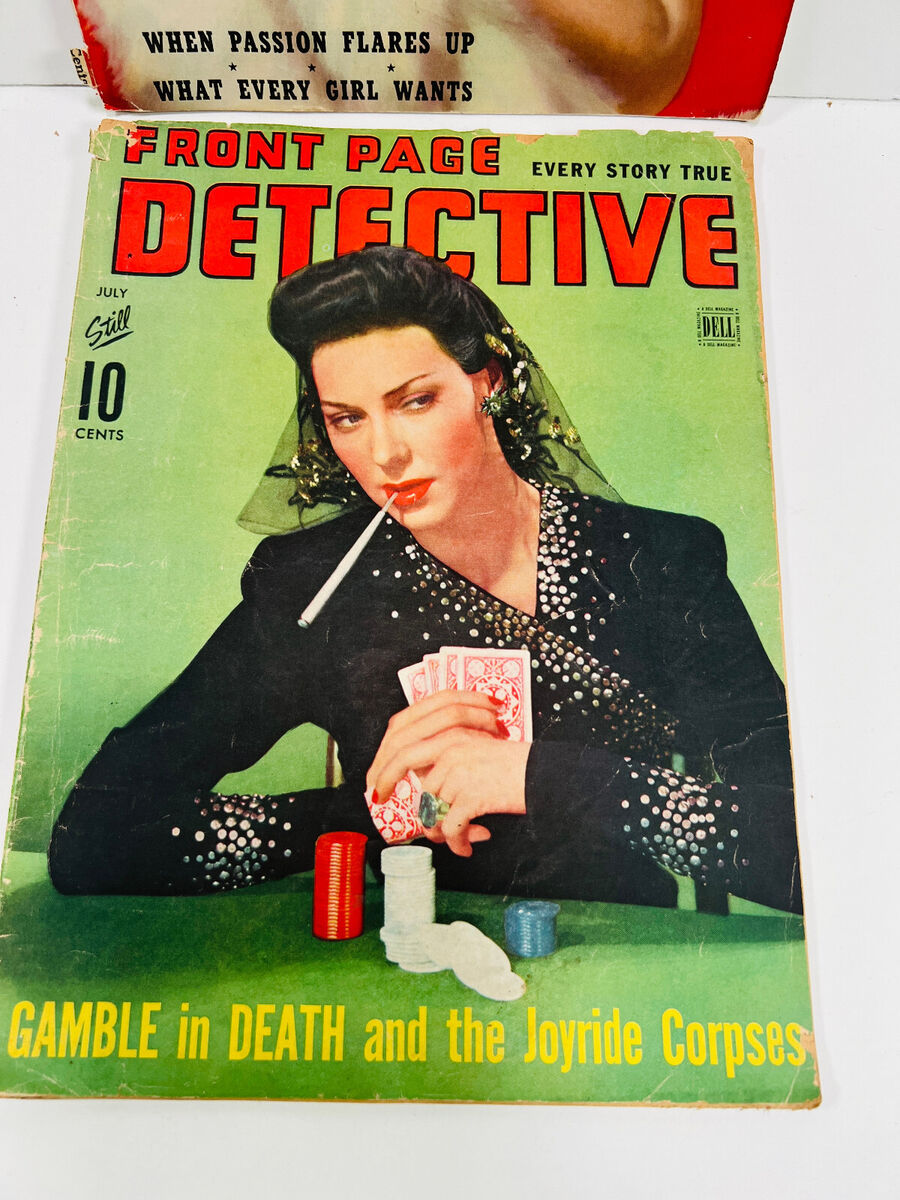This image captures an old, worn magazine cover with distinctive features. The cover, which appears to be light green, sports the bold red title "Front Page Detective" at the top, with the black tagline "Every Story True" next to it. Below that, it is noted that the issue is from July and priced at 10 cents, marked in black text. The central figure on the cover is a woman dressed in black with intricate, shiny adornments on her sleeves and collar. She has dark hair, a black veil pulled back from her head, and is wearing red lipstick. A long cigarette holder dangles from her mouth, and she holds red playing cards close to her chest. In front of her, on a green felt table, are stacks of poker chips in red, white, and blue. Her right elbow rests on the table, adding to her contemplative, engaged posture. At the bottom of the cover, in yellow letters, the text reads "Gamble in Death and the Joyride Corpses." Visible behind this cover is another red poster with partially obscured text in black that reads, "When Passion Flares Up, What Every Girl Wants," hinting at its placement beneath the featured magazine on display.